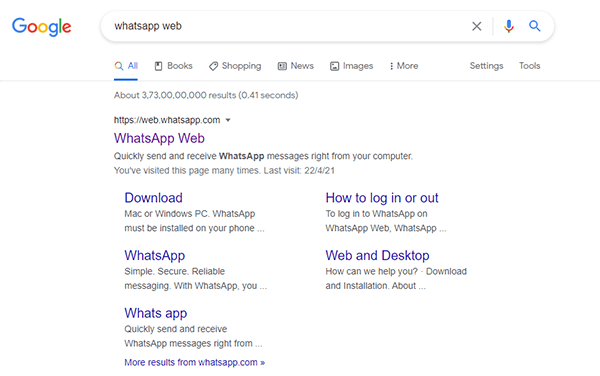Screenshot of a Google Search Results Page for "WhatsApp Web"

The image is a screenshot taken from a website, set against a white backdrop. In the upper left-hand corner, the colorful Google logo is prominently displayed: the first "G" appears in blue, followed by the first "O" in red, the second "O" in yellow, the "G" again in blue, the "L" in green, and the final "E" in red. To the right of the logo is the Google search bar, containing the query "WhatsApp web" written in black text.

Below the search bar, a navigation menu appears, listing various categories in black text: "All," "Books," "Shopping," "News," "Images," "More," "Settings," and "Tools." Just below this menu, the search results are summarized, indicating about 3,730,000,000 results found in 0.41 seconds.

The first search result displayed features the URL "https://web.whatsapp.com" in black text, with the title "WhatsApp Web" in purple. A brief description below this reads, "Quickly send and receive WhatsApp messages right from your computer. You visited this page many times. Last visit: 21-4-21." Below this description, there are several blue hyperlinks: "Download," "WhatsApp," "WhatsApp," and "How to log in or out." Further down, there is a section labeled "Web and Desktop."